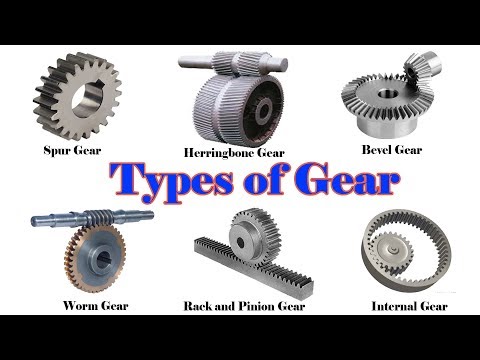The image depicts six metal gears arranged on a white background, with three gears on the top row and three on the bottom row. In the center, between the two rows, the phrase "Types of Gear" is prominently displayed in blue text. Each gear is labeled: starting from the top left, there is a spur gear which resembles a round bolt or tire, followed by a herringbone gear, which looks like two interlocking gears or a tire with a pipe on top. Next, there's a bevel gear, which has a conical appearance similar to a chef's hat. On the bottom row, from left to right, we see a worm gear that resembles a bolt with a long bar or a circle hanging from a pipe, followed by a rack and pinion gear, featuring a gear rolling on a horizontal path, and finally, an internal gear which consists of a smaller gear enclosed within a larger circle. The image also includes black horizontal bars at the top and bottom, framing the arrangement of the gears.